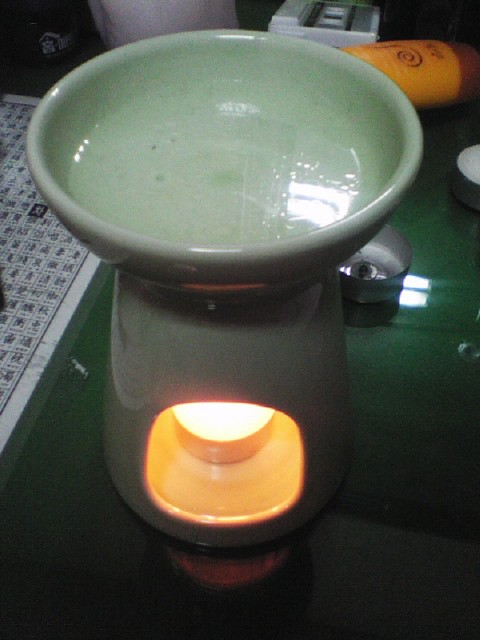The full-color indoor photograph features a jade green ceramic burner, designed to hold a tea candle in its base, with a small green bowl on top likely containing liquid or potpourri. The green burner sits on a matching green table or countertop. To the upper right, there is an orange tube-like object and a used-up tea candle with a burnt wick. To the far left, a white mat with green inlay is partially visible, and a gray object is discernible in the background. The overall scene is detailed and cohesive with repeated emphasis on the green hues and the presence of various surrounding objects.